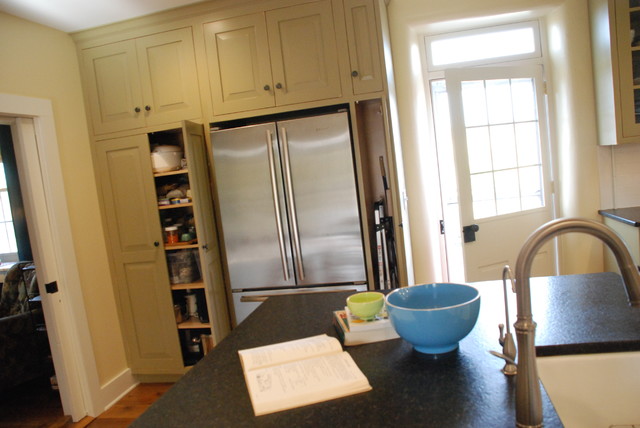This detailed photograph of a kitchen, taken during the daytime, captures a well-lit space filled with kitchen essentials. Central to the image is a large, silver stainless steel refrigerator with a two-door top section and a bottom drawer, complete with both vertical and horizontal silver handles. To the refrigerator's left, a tall pantry with two open doors reveals items neatly arranged on six shelves.

Adjacent to this pantry is an open entryway leading into another sunlit room, highlighting the inviting and airy ambiance of the home. Towards the right of the refrigerator, along the back wall, is a distinctive door with a nine-paned window at the top, partially open to allow bright, natural light to pour into the kitchen. The door and its frame are painted a soft yellowish beige, and the window includes a top rectangular section that appears operable.

In the foreground, spanning from the lower right corner to three-quarters across the frame, an L-shaped kitchen countertop is prominent. This dark grayish-brown countertop features a white sink with a sleek, silver faucet arching gracefully over it. Resting on the counter are a blue bowl and a couple of books, one of which is open, hinting at an interrupted moment of casual reading or perhaps a recipe in progress. A green bowl sits atop the stacked books, adding a small but vibrant touch to the serene kitchen scene.